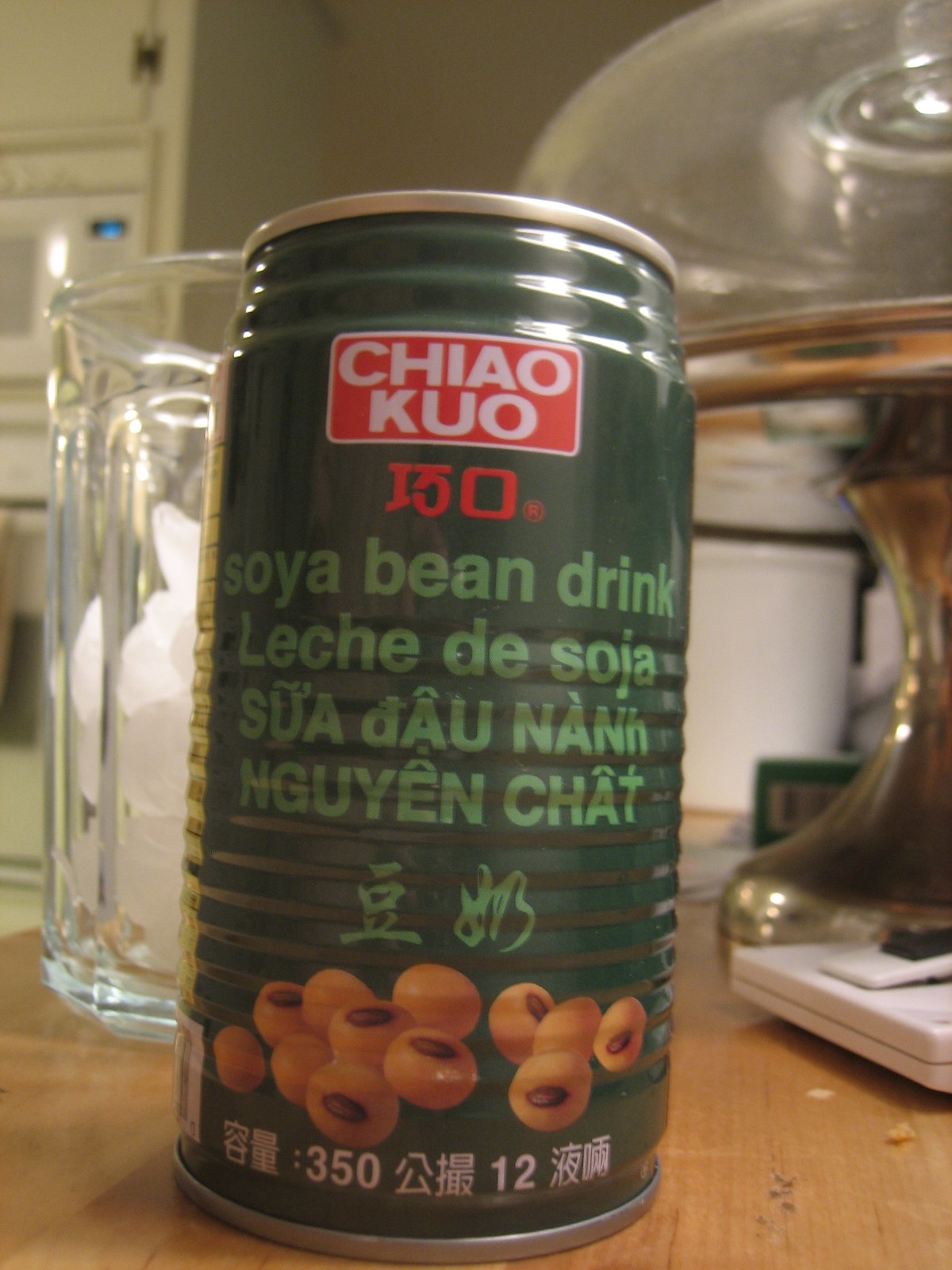A detailed caption for the image:

"A vibrant green can of soybean drink is prominently featured in the foreground of this photo, characterized by its Asian script at the bottom. Behind the can, a clear glass filled with ice is positioned, adding a refreshing element to the scene. To the right of the drink, a brass cake stand with an elegant clear glass dome presents a sophisticated contrast. In the background to the left, a long cabinet with upper doors is visible, housing a microwave oven with distinctive blue lights and a digital timer display. The setting is completed by a wooden table surface and a white object situated on the right edge of the image."